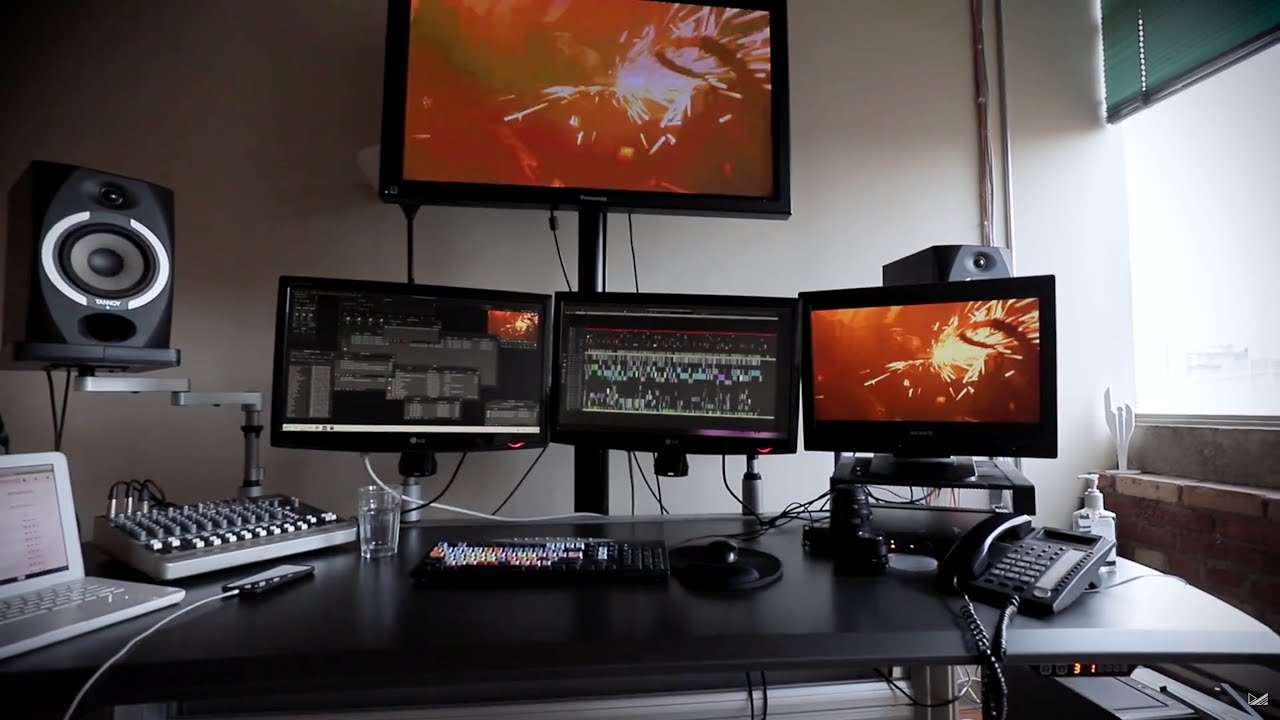This detailed image showcases a sophisticated indoor computer workstation, illuminated by daylight streaming through an open window on the right side of a white wall. The black desk is equipped with three neatly organized computer monitors positioned in a row on stands, each displaying different content: the left showing gray boxes with white text, the center depicting colorful bars typical of editing software, and the right displaying an orange and black scene with a burst of sparks, mirrored on a larger top monitor, suggesting an industrial setting.

Above these screens, a significantly larger monitor echoes the image from the rightmost screen, further highlighting the dramatic burst of sparks. On the left side of the desk, a white open laptop sits adjacent to a device described as a mixing box, connected with various cords. Above, black speakers mounted on floating shelves or small stands flank the monitors, hinting at the high-quality sound setup. A cell phone connected by a white cord rests nearby.

On the right side of the desk, practical items like a black office landline phone and a bottle of hand sanitizer signify the blend of professional and personal use of this space. The desk also features a keyboard with multicolored keys, a mouse on a pad, and a glass of water, indicating ongoing and detailed work, possibly in music, video editing, or other multimedia tasks. High on the right wall, a window brings natural light into the room, and a small platform holds a cactus, adding a touch of greenery to this well-equipped technical environment.